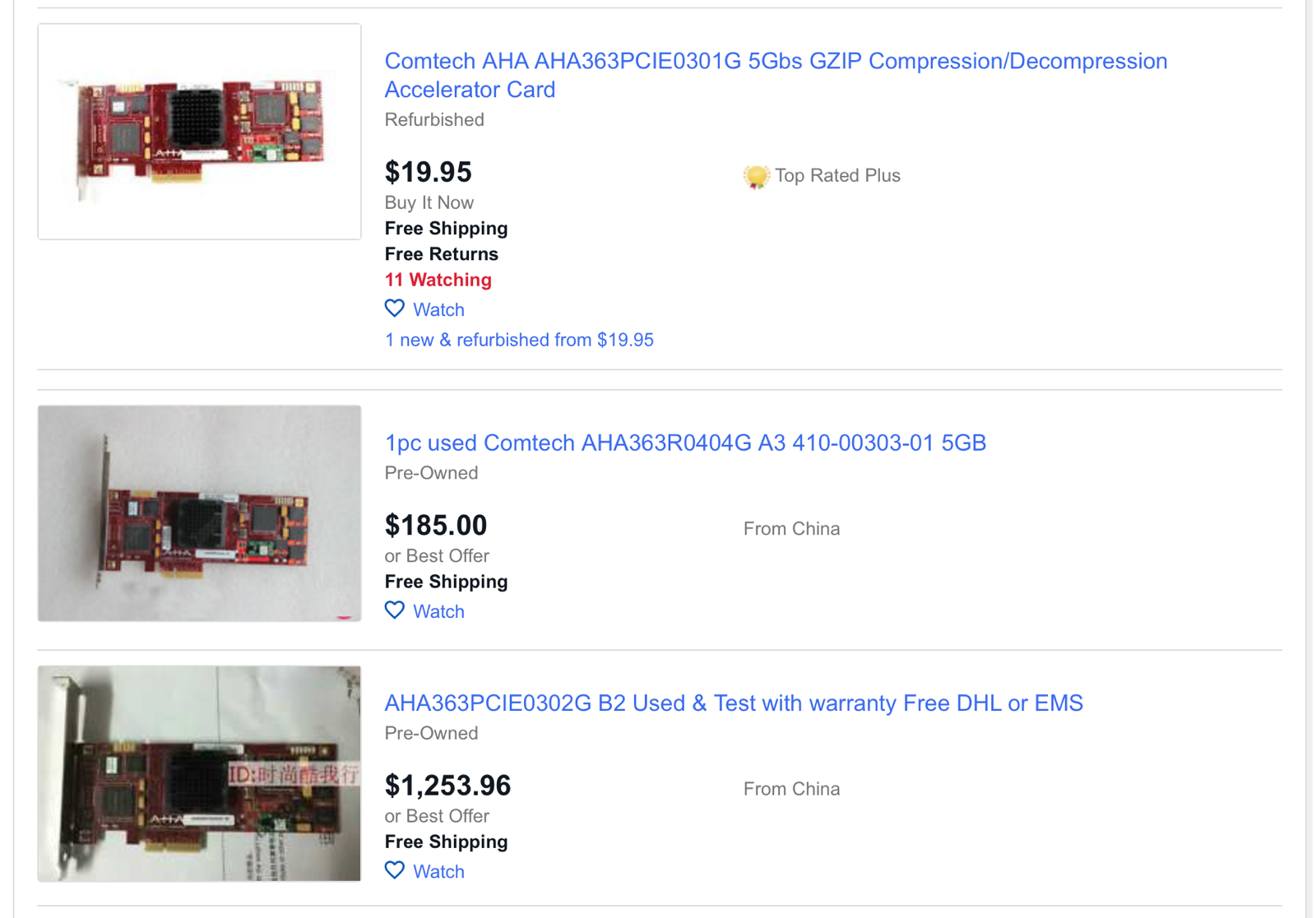**Detailed Caption:**
Comtac AHA-363 PC-0301G 5GB G-Zip Compression and Decompression Accelerator Card, Refurbished in 1995. Available for purchase now with free shipping and free returns. Currently, 11 users are watching this item with a "Buy It Now" price option. This product is top-rated and categorized as a single piece. Additionally, there are options for both new and refurbished units from 1995.

Another listed item is the Comtac AHA-363-R0404G-A3-410-00303-015GB, which is pre-owned and available for $185 or best offer, shipping from China with free shipping included. There is also a Comtac AHA-363 PC-302G-B2 model, used and tested with a warranty, priced at $1,253.96. This unit also ships from China with free DHL or EMS shipping. Multiple listings for the AHA-363 PC-302G-B2 model are available at the same price, all offering free shipping via DHL or EMS and accepting best offers.